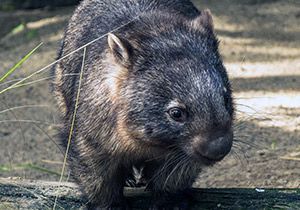This is an up-close photograph of a mammal, possibly a rodent like a squirrel. The animal is situated in an outdoor setting, standing on the ground with noticeable elements like dirt and a few blades of green grass on the left side of the image. Shadows from the light play across the scene. The photograph captures the creature head-on, although the head is slightly turned to the right, revealing part of its body but not its tail. 

The animal exhibits a blend of colors—black, brown, gray, and tan with some white and beige markings. Its fur includes various patches: a lighter patch near the right ear, white and silver markings on its back, and a white edge on the pointed, upright ears, which are darker on the outside. The creature has small dark brown eyes and distinctive whiskers under its nose. Additionally, its face shows a mix of black and white coloring. It stands robustly, with one paw appearing to rest in front of a limb, adding to the natural and dynamic composition of the photograph.